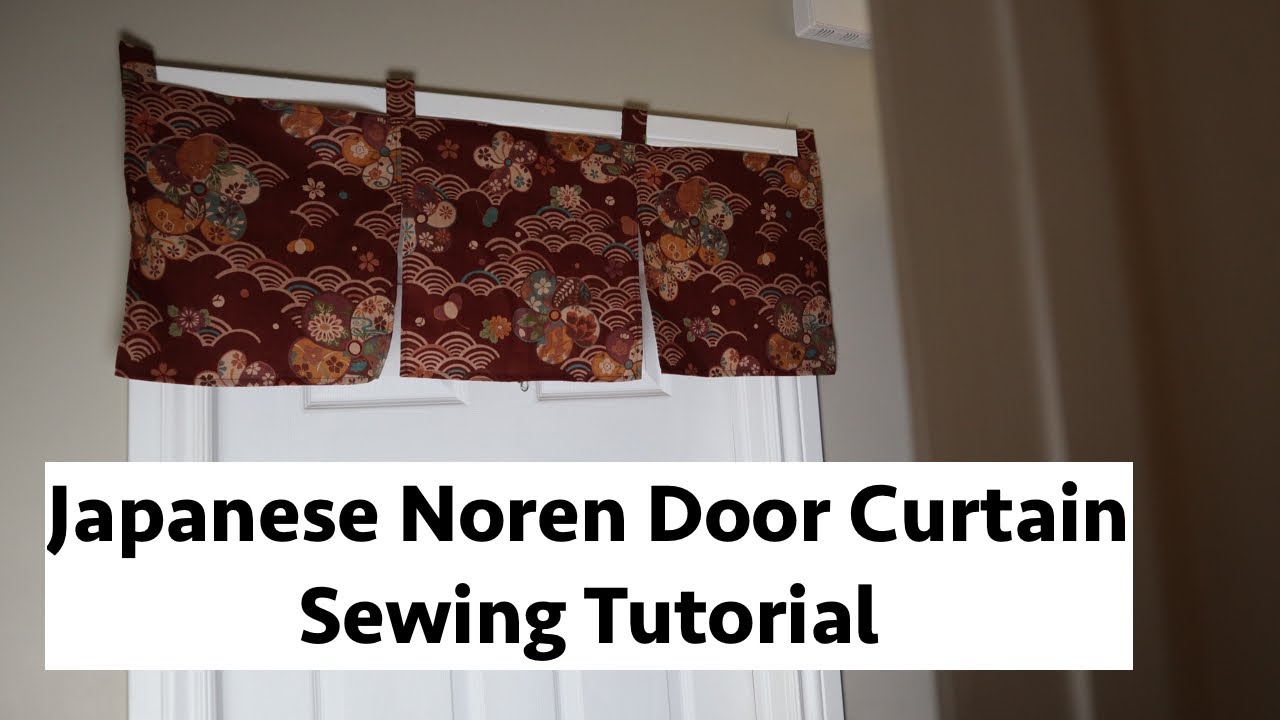The image depicts an indoor scene of a room featuring a white door centered within a white doorframe, set against a beige wall with dark shadows on the right side. Above the door hangs a set of three small maroon Noren door curtains, emblazoned with colorful Japanese fan designs in red, green, and orange hues. The curtains appear to be placed for display purposes, consistent with a sewing tutorial theme. At the bottom of the image, bold black text on a white background reads, "Japanese Noren Door Curtain Sewing Tutorial." The scene also includes a smoke detector mounted at the top right corner of the wall, adding to the domestic setting.